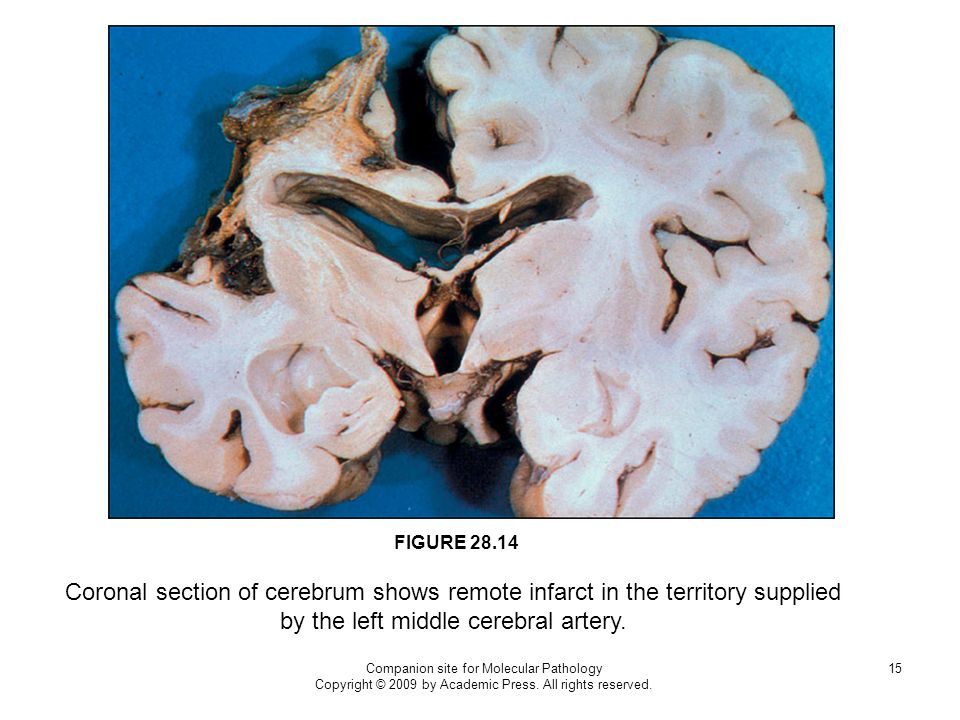The image presented is a detailed photograph of a coronal section of the cerebrum, showcasing a remote infarct in the territory supplied by the left middle cerebral artery. The photograph, featuring a cross-section of the brain with characteristic warbly, brain-like structures and central voids, is set against a blue background. The image is labeled as "Figure 28.14," and beneath it, a secondary description repeats: "Coronal Section of Cerebrum Shows Remote Infarct in the Territory Supplied by the Left Middle Cerebral Artery." Further description includes smaller text reading, "Companion Site for Molecular Pathology, Copyright 2009 by Academic Press, All Rights Reserved," indicating the source as a scientific publication likely from a textbook or journal titled "Molecular Pathology." The number 15 is located in the lower right-hand corner, possibly signifying a page number or slide reference. The model of the brain appears to be photographed in meticulous detail, bringing attention to the infarct area with a mix of white and pinkish hues around the edges.